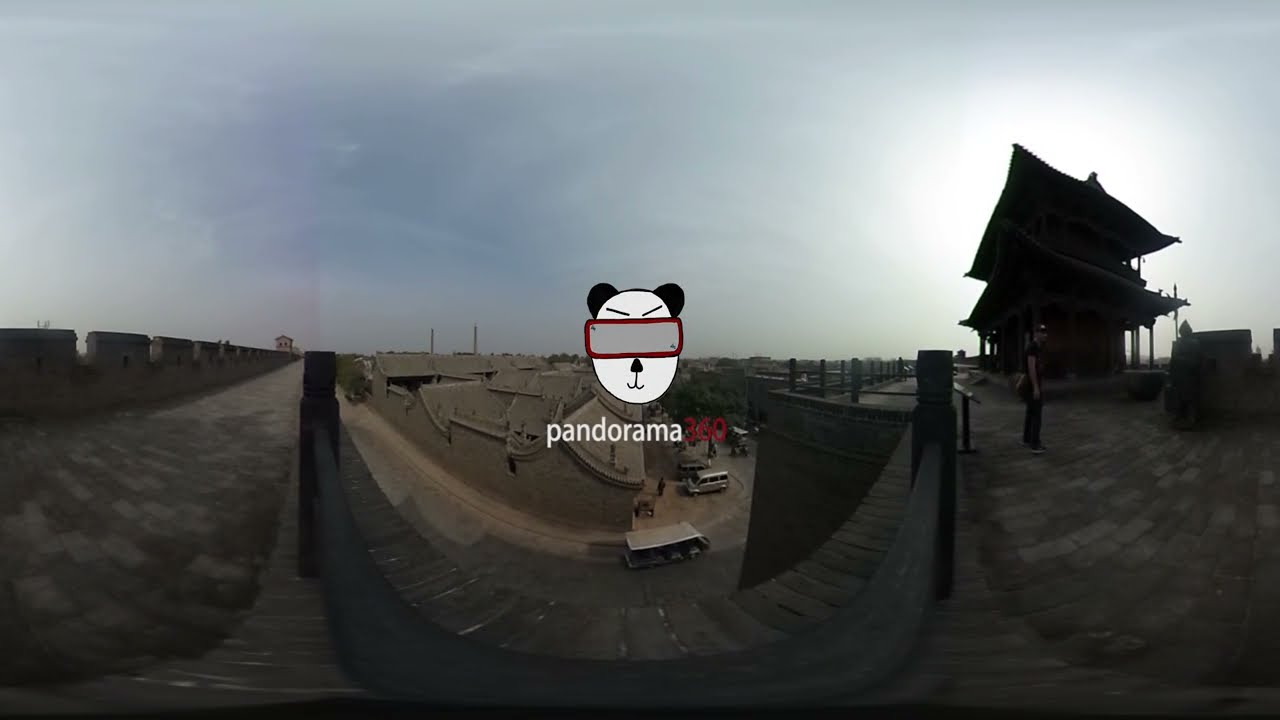This panoramic image, possibly taken at dusk, captures the historic Pingyao Ancient City Walls in China. The photograph, distorted due to its panoramic nature, offers an expansive view from a vantage point atop the tall, wide brick walls, which are reinforced with turrets and feature wooden railings. Below, the scene shows both dusty farmland and an assortment of buildings, hinting at a lived-in area with homes or businesses. To the right stands a distinctive two-story traditional Chinese building, constructed from wood and adorned with double-tiered, pointed roofs typical of ancient Asian architecture. A person dressed in all black, with a bag and black baseball cap, can be seen walking away from the camera near this building. Overlaying the center of the image is a logo of a cartoon panda bear with a gray bar over its eyes, accompanied by the text "Pingyao Ancient City Walls, Pingyao" in English, with additional text in red and white Chinese characters below. The sky is hazy with clouds but retains some patches of blue, complementing the historical and serene atmosphere of the vista.